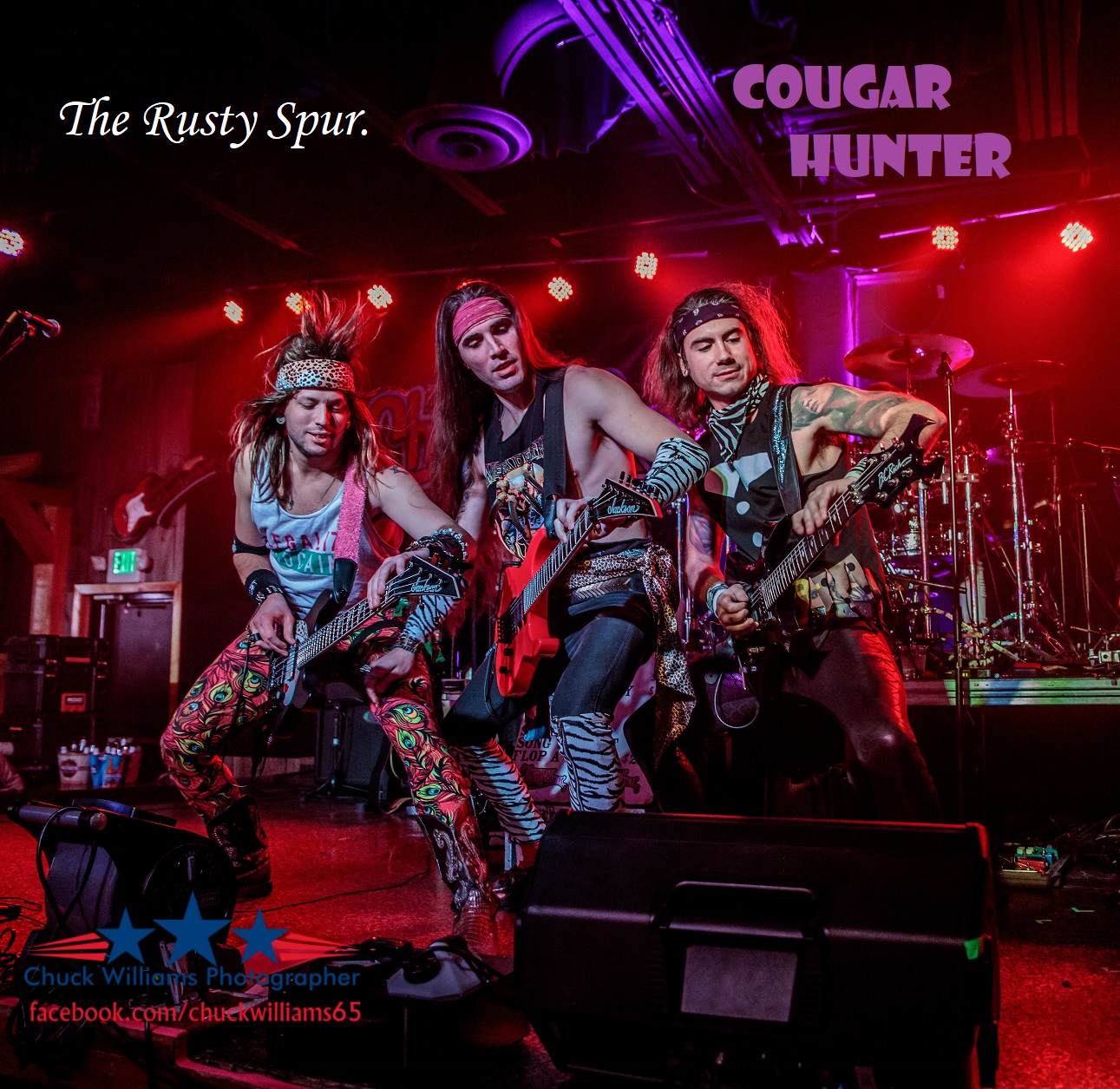The poster is a square-shaped photograph capturing a vibrant concert scene featuring three musicians on stage. All three, dressed reminiscent of a 70s or 80s rock band with long hair, headbands, ripped tank tops adorned with zebra and cheetah prints, tight pants, and boots, are energetically playing electric guitars or bass. The musician on the left stands out with his spiky blonde hair and cheetah print headband. The stage is bathed in intense red lighting, highlighting various instruments, including a drum set, and accompanied by speakers. An exit sign with a door is visible on the mid-left side. At the top-left corner of the poster, the name "The Rusty Spur" is prominently written in white lettering, while "Cougar Hunter" is displayed in light purple on the top-right. The bottom left corner credits Chuck Williams as the photographer, followed by three blue stars and the text "facebook.com/ChuckWilliams65".